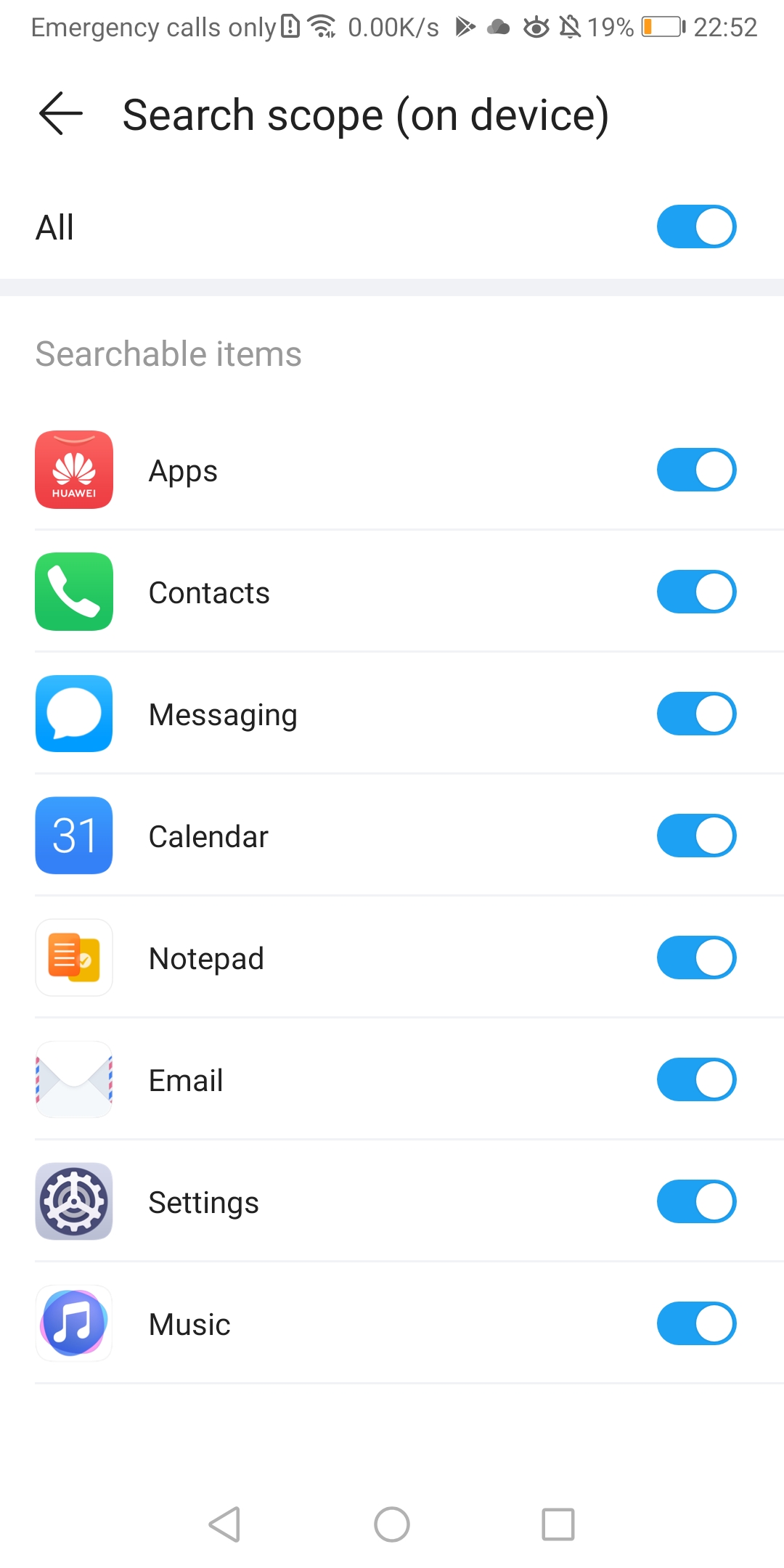A detailed screenshot of a smartphone screen displays the device's user interface at 10:52 p.m., with a battery level of 19% indicated in the top right corner. Directly beneath the time and battery status, the title "Search Scope" is prominently displayed, suggesting it is the current view or feature in use. Below this title, a list is labeled "Searchable Items," each accompanied by a blue toggle switch positioned to the right, indicating they are enabled for search functionality.

The list of searchable items includes various categories such as Apps, Contacts, Messaging, Calendar, Notepad, Email, Settings, and Music. This configuration implies that the user can search for information across these categories using a unified search feature, likely referred to as "Search Scope." This could be a search bar found within the app menu or a similar interface, enabling the user to quickly find relevant content across multiple applications by simply typing in a query.